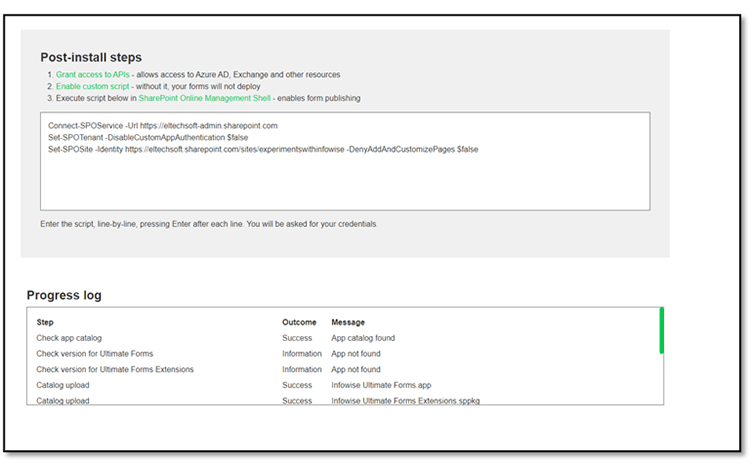**Post-Installation Steps Interface for SharePoint Online Forms Deployment**

The image depicts a detailed "Post Installation Steps" page pivotal for deploying custom SharePoint Online forms. 

1. **Grant Access to APIs**: This step ensures that permissions are correctly set up to allow access to critical resources like Azure Active Directory (Azure AD), Exchange, and other integrated services crucial for the operation of your forms.
   
2. **Enable Custom Script**: Highlighted next is the necessity to enable custom scripting on your SharePoint environment without which the forms will not deploy. This is a critical step for the functionality of custom forms.
   
3. **Execute Script Below**: Users are instructed to run the provided script using the SharePoint Online Management Shell to enable form publishing. An accompanying text box contains the script, with a note advising users to enter the script line by line, pressing enter after each line. During execution, credential prompts will appear, necessitating user authentication.

Additionally, the bottom of the page has a "Progress Log" section, documenting the checkpoints in the script execution process. The log outlines the following:
- **Check App Catalog:** Success
- **Check Version:** Repeatedly notes "app not found"
- **Catalog Upload Success:** Indicates positive confirmation of uploads.

The overall context explains scripts as batch instructions executed by a computer to automate tasks, making the deployment process smoother and more efficient. The three lines of commands in the script are specific to SharePoint functions.

This interface is designed to guide users through the precise steps necessary to ensure the smooth deployment and operation of custom forms within SharePoint Online.